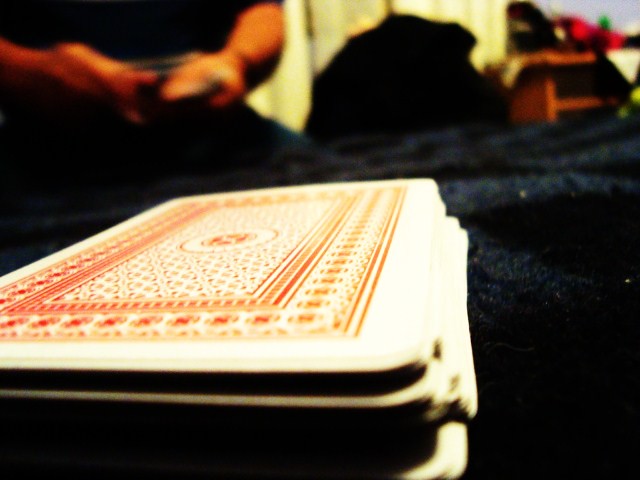In this detailed close-up image, a deck of playing cards lies atop a dark blue sheet that is noticeably wrinkled and folded. The deck is positioned in the bottom left-hand corner, stretching towards the center. The top card, like the rest of the deck, features a white border encasing an intricate red design. The design includes a border of parallel red lines, various geometric patterns, another series of geometric red lines, and a central red circle filled with more red coloration.

In the upper left-hand corner, the blurry shape of a person kneeling is visible. This person is dressed in a black shirt and blue pants, with a medium skin tone. The top right-hand corner also has a blurry background, showing a wooden shelf with two layers. The shelf holds several objects, including red, white, and black items. Adjacent to the shelf is a bulky, lumpy black object. Behind all these elements, white blinds can be faintly seen.